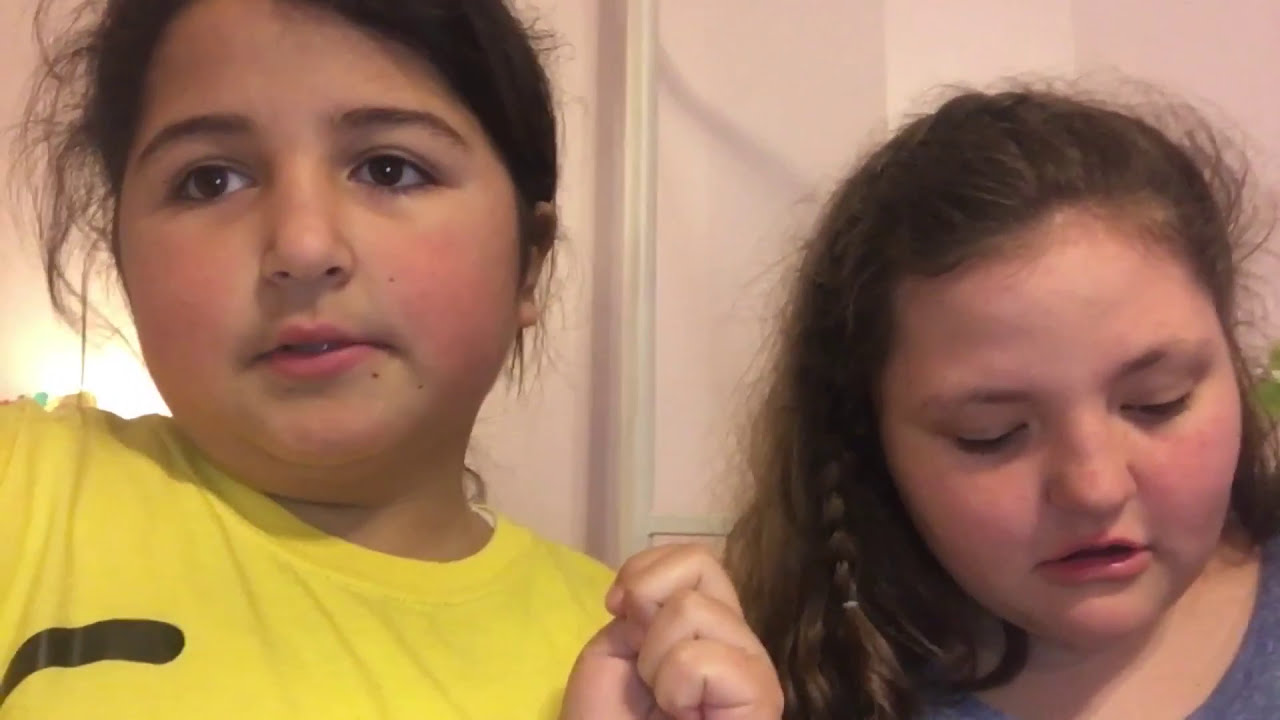This photograph captures two young girls standing side by side in an indoor setting with a white background. The girl on the left has dark hair and wears a yellow t-shirt featuring a black design. Her left hand is raised in a fist, and she gazes forward, slightly over the left shoulder of the camera. Behind her right shoulder, a light source is visible, casting a gentle glow. The girl on the right, slightly shorter, has brown hair styled with a front braid and wears a blue shirt. She is looking downward, giving the impression she might be speaking. Despite minor shadows and details like a small pole along the wall, the overall scene is simple with no text, focusing on the candid moment between the two girls who appear to be of grade school age.